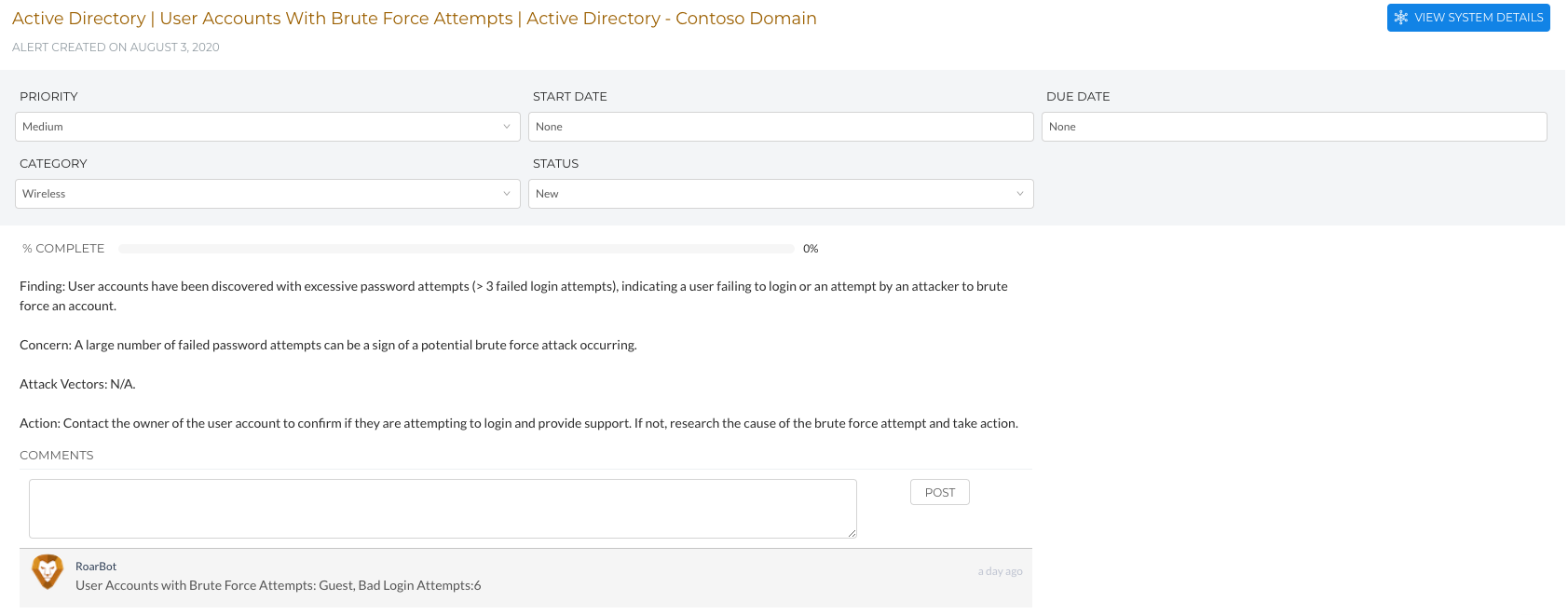This detailed caption provides context for a screenshot taken from a digital device, likely depicting either a computer website or an application interface. The screenshot is significantly zoomed out, rendering the text nearly illegible. 

In the top left corner, highlighted in orange font, the screen specifies "Active Directory User Accounts with Brute Force Attempts Active Directory Contasso Domain." On the upper right side, there's a blue rectangle button featuring a white star logo, labeled "New System Details." 

Further down, the webpage showcases four dropdown menus or text boxes designed for information input, each labeled with titles too minute to discern. These elements are set against a subtly off-white or grayish background.

Beneath this section, the background transitions to white, with some black text inscribed on it, although the text remains indistinct due to its minuscule size. At the very bottom, there's a white text box accompanied by an adjacent "Post" button.